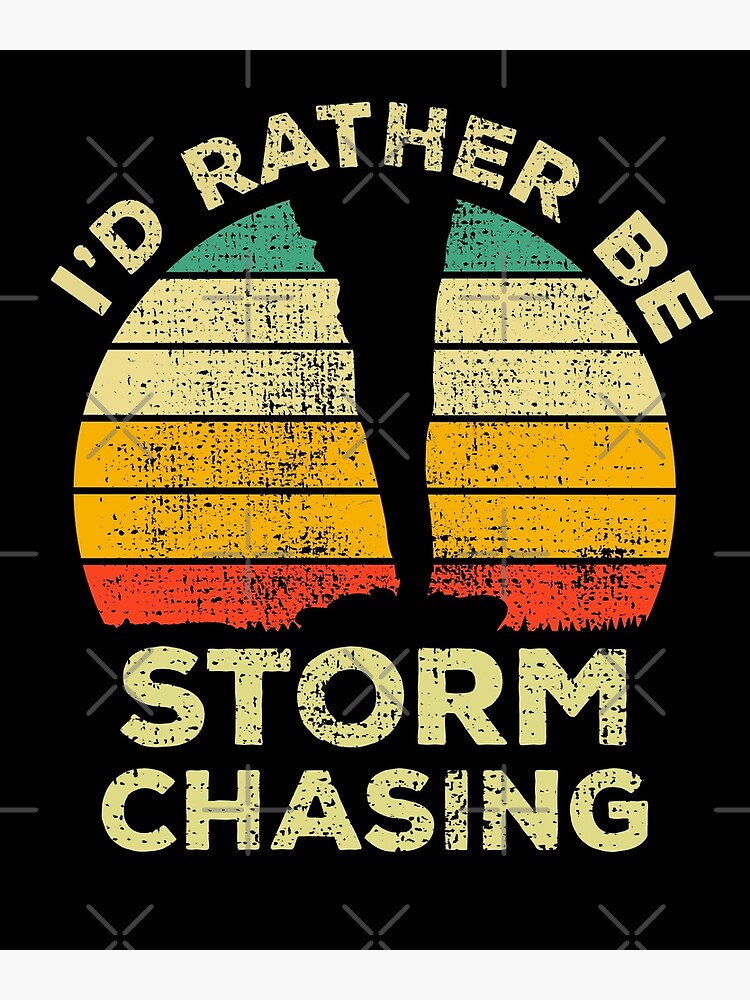This graphic illustration, evocative of a vintage poster, prominently features a central circle adorned with alternating stripes in hues of red, yellow, off-white, and aqua. Cutting through the middle of this circle is the striking silhouette of a tornado, its funnel descending dramatically. Encircling the top of this graphic element, the phrase "I'd rather be" appears in block text, arcing clockwise around the upper perimeter. Similarly, the words "storm chasing" stretch horizontally beneath the circle, balancing the composition. Both texts exhibit a weathered, rubbed texture, enhancing the design with a nostalgic, worn look. The background is rendered in flat black, intersected subtly by small gray Xs and horizontal lines that quarter the image, adding depth and structure to the overall design.